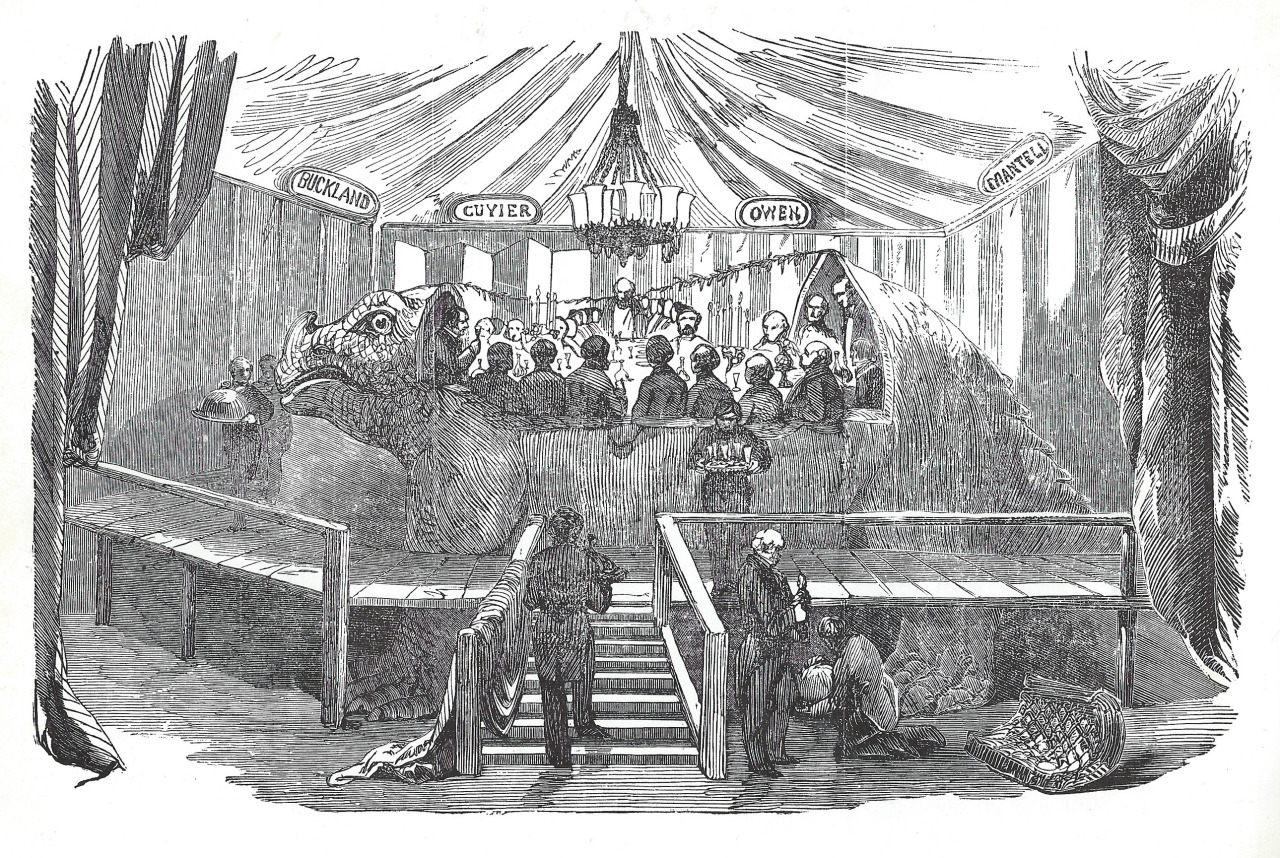The image is an old-fashioned, meticulously detailed black and white line drawing, created using only simple pen strokes. It takes place inside a black and white striped circus pavilion. The ceiling curves upwards, centrally adorned with a large chandelier. Underneath this chandelier, on a raised wooden platform supported by multiple legs, sits a large cutout of a lizard-like dinosaur, which serves as an unusual dining area. Numerous men are seated inside this dinosaur cutout, engaged in a meeting while dining. Serving attendants carrying food platters and drinks are moving towards the platform, navigating steps to reach the diners. The scene includes names like Buckland, Cuvier, Owen, and Mantel inscribed at the top. The entire composition exudes a sense of antiquity, evoking a setting reminiscent of the 1900s, reflected in the clothing and the meticulous pen and ink style.